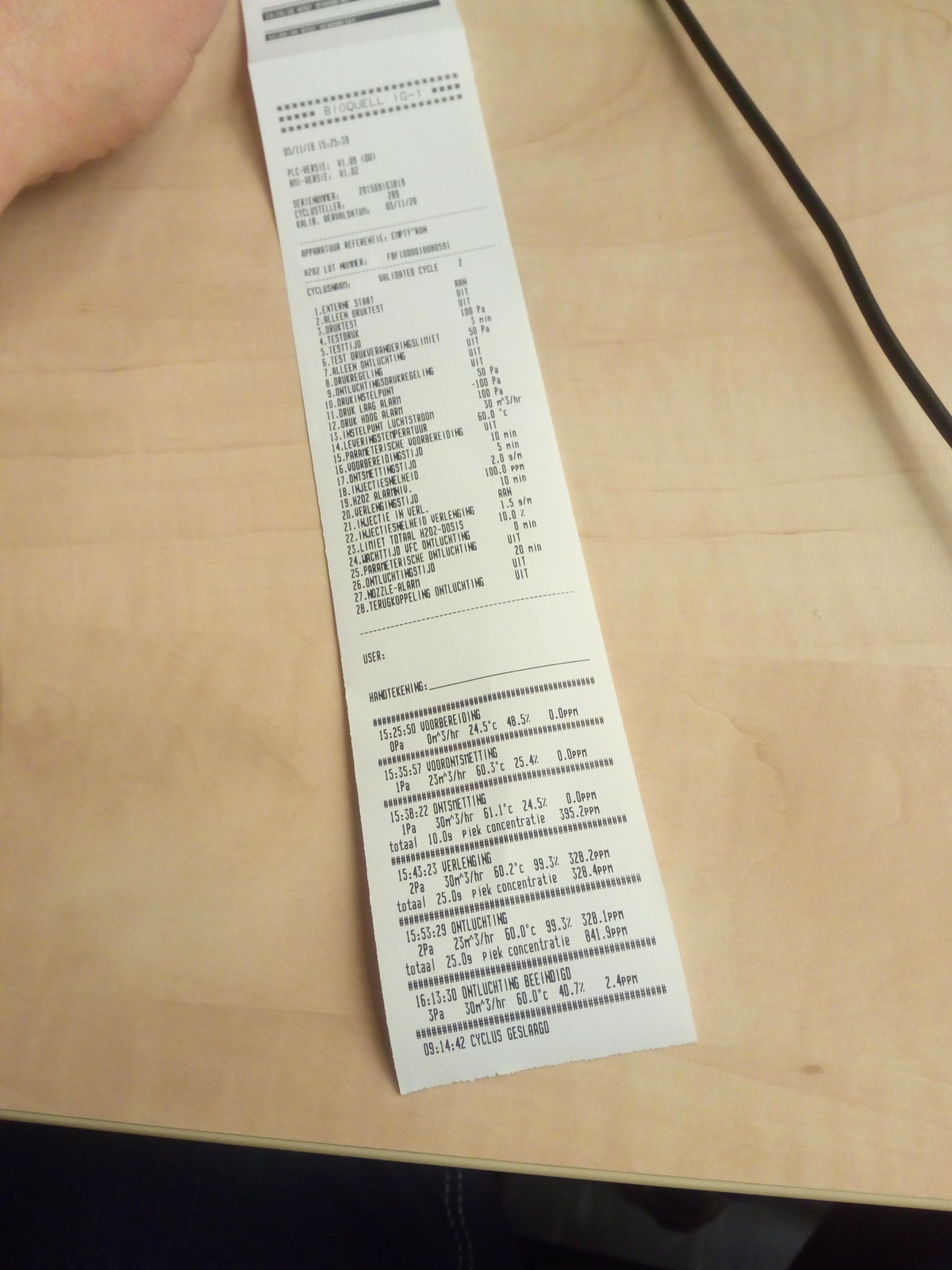A detailed photograph captures a thin, long receipt resting on what appears to be a wooden surface. A power cord is partially visible in the upper right-hand corner of the image, while a human hand intrudes into the frame from the upper left corner. The receipt is printed on white paper and lists approximately 28 items. Unfortunately, the text on the receipt is somewhat blurry and difficult to read, especially towards the top, which is further obscured by the camera angle. The text itself might not be in English, possibly German, though this is not definitively clear. The overall impression leaves some ambiguity as to whether the document is, in fact, a conventional receipt or some other type of printed item list.